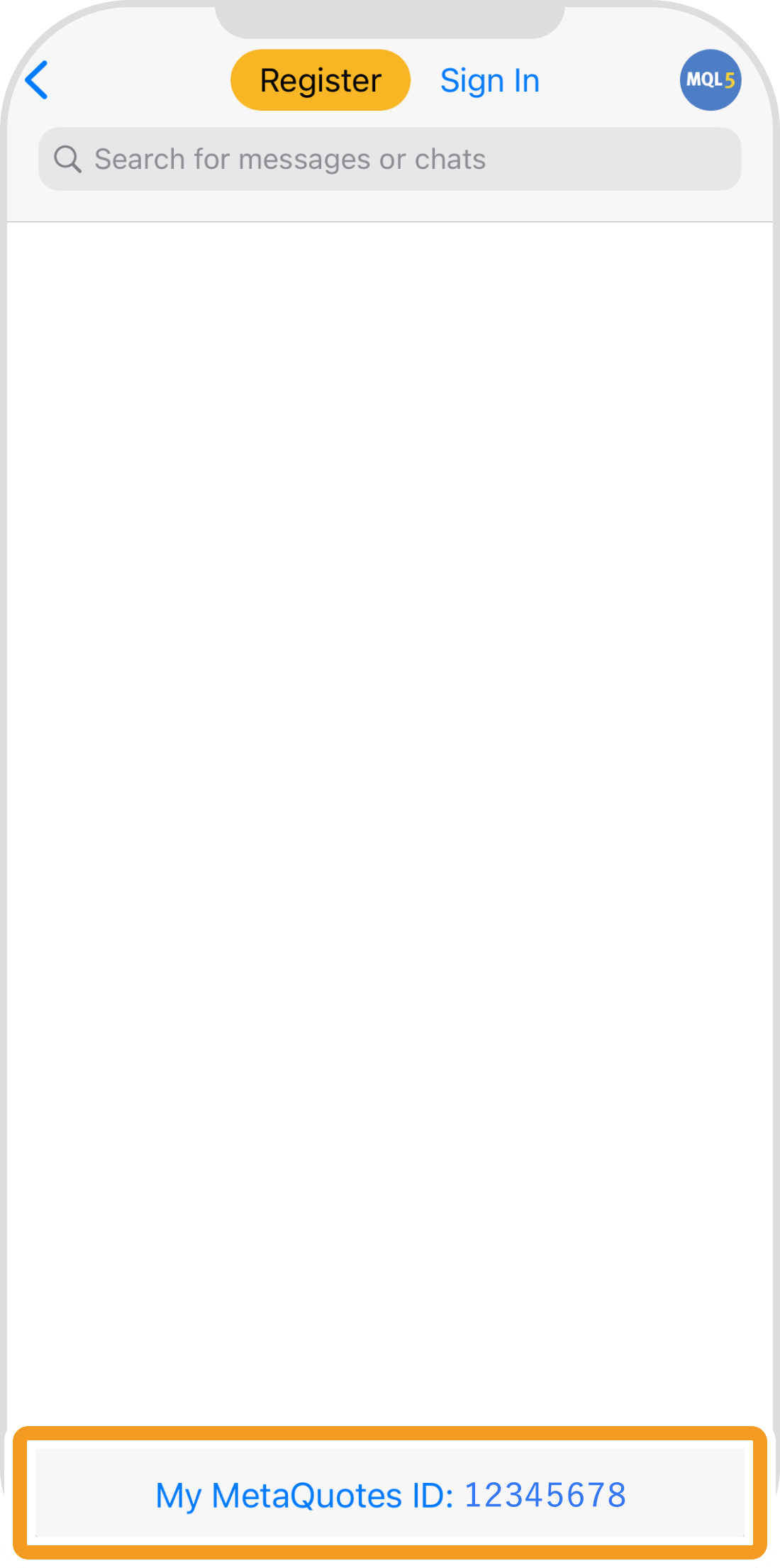### Caption:

This mobile screenshot appears to be a mock-up for a mobile app. In the upper-left corner, there's a blue, left-facing chevron arrow. Toward the center-left of the screen, there’s a yellow, pill-shaped button with black text that reads "Register." Next to this button, slightly to the right, is blue text that says "Sign In," with both 'S' and 'I' capitalized. Further right, there's a blue circle containing the white text "MQL" and a yellow number "5."

Below these elements lies a search bar featuring the placeholder text "Search for Messages or Chats," preceded by a magnifying glass icon. The majority of the screen is blank, showcasing a plain white background. Near the very bottom, enclosed in an orange-outlined square with a light gray background, is blue text that reads "MyMetaQuotes," with the 'M' and 'Q' capitalized. Additionally, it includes "MyMetaQuotesID: 0AB00C00."